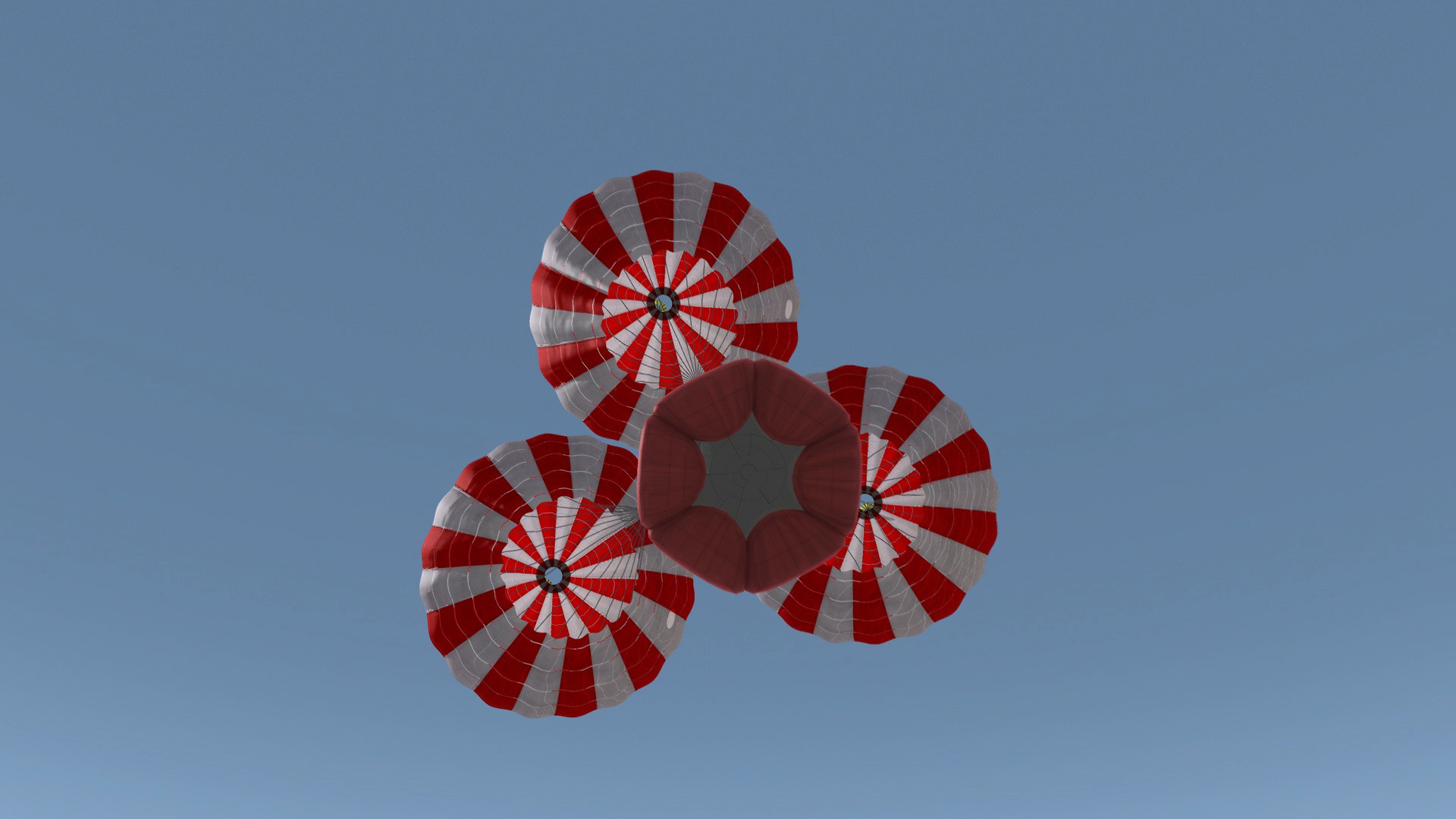The image depicts a vibrant, daytime scene captured from the ground, looking directly up at the sky. The sky has a bluish-gray tint, providing a striking backdrop for the primary subjects. Dominating the middle of the photograph are four hot air balloons, each with unique patterns. One hot air balloon is almost a solid red color, distinguished by a diamond pattern visible on its underside. Surrounding this central balloon are three others, each adorned with red and white stripes that converge into a point at their black tops. Notably, three parachutes are also present in the scene, slowly lowering an unseen object towards the ground, possibly something from a satellite or a spaceship based on the configuration of the parachutes, suggesting a careful descent. The photograph captures a moment of serene yet dynamic activity in the sky, blending human engineering marvels with the tranquility of hot air ballooning.